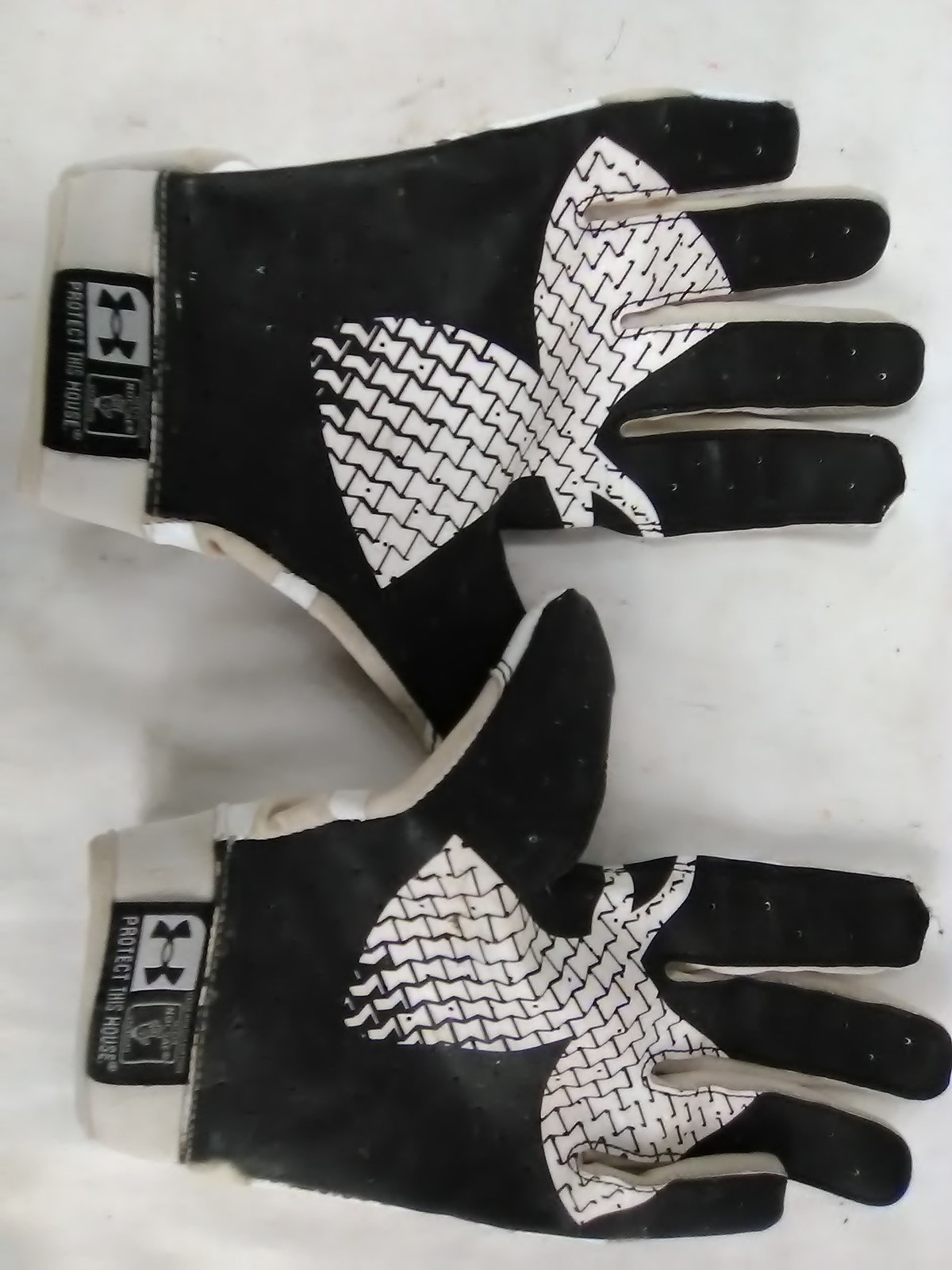This image showcases a pair of used riding gloves arranged with the palms open and facing the viewer, displayed against a white background. The gloves, predominantly black with a striking white design, are from the Under Armour brand. Each glove’s palm features an alternating hourglass-shaped pattern in white, which forms a stylized version of the Under Armour logo when the gloves are placed side by side. The wrists of the gloves bear a black and white tag that includes the Under Armour logo and the phrase "Protect This House." The logo is also prominently displayed on the wrist area of the gloves. These gloves, which could be used for motorcycle riding or other sports, appear to be made of a good quality leather material.